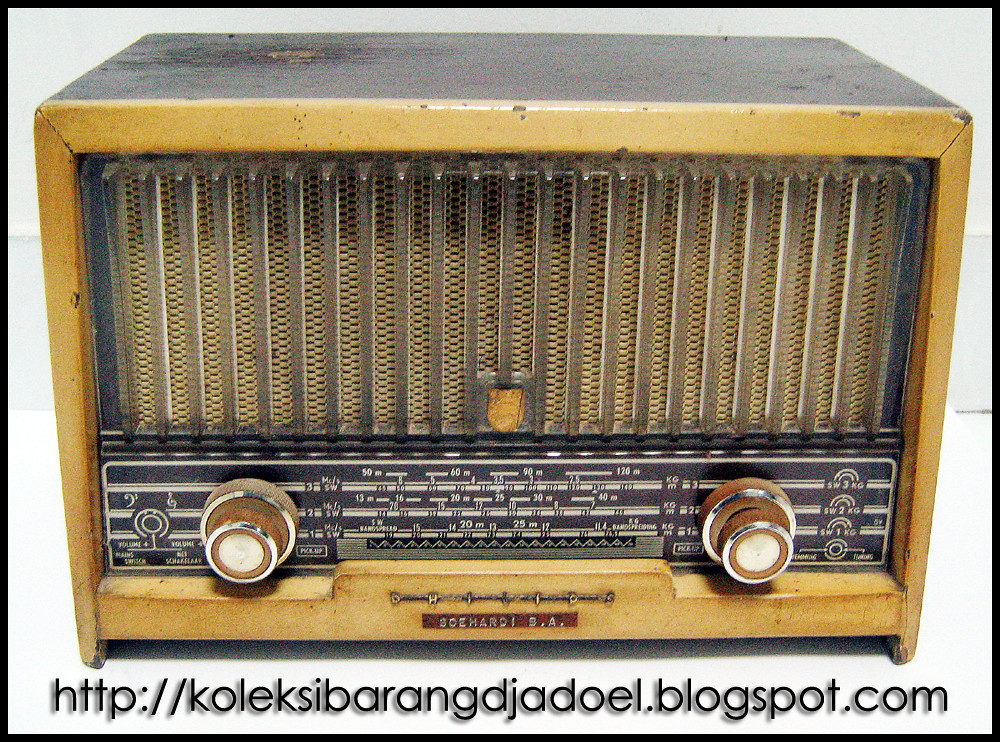The photo captures a vintage Kolsky brand radio, displaying noticeable signs of aging with its rusted and weathered appearance. The radio's body features a combination of light and dark brown hues, with a top section in black wood. It is equipped with two knobs, one on each side of the central black display, which lists various frequencies in white letters, including 50, 60, 90, and 120. At the bottom of the picture, the text "http://koleksibarangdjadol.blogspot.com" is visible, framed by a black border. The background transitions from white to off-white, accentuating the antiquated charm of the radio, suggesting it has likely been stored away for many years.